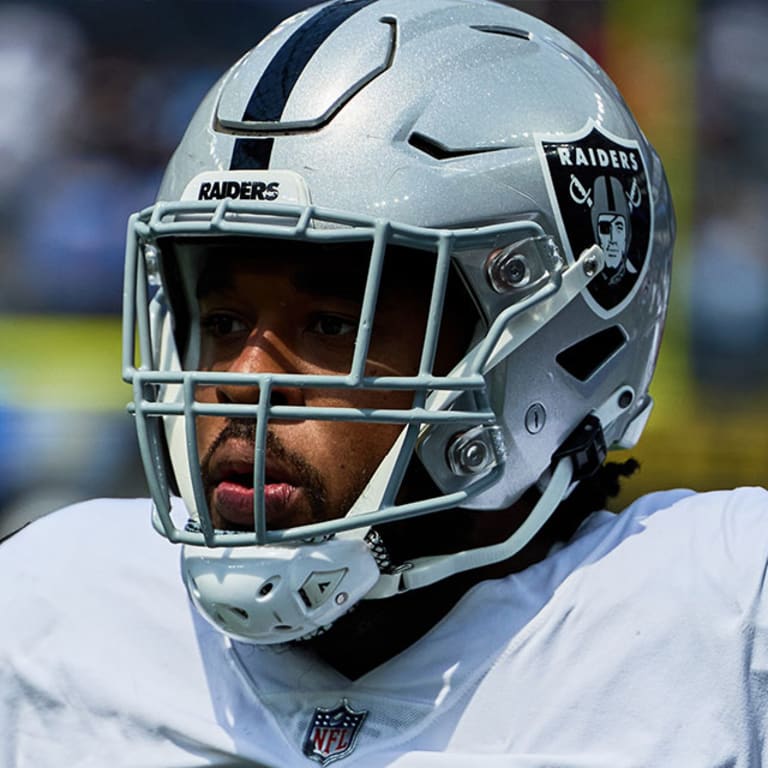The image features a clear, close-up view of an NFL football player from the shoulders up, focusing primarily on his helmeted face. The player, who appears to be a Black man with dark facial hair and a slight mustache, wears a silver and black Raiders helmet prominently displaying the team's logo—a man with an eyepatch and crossed swords. The helmet also features a black stripe down the middle with the name "Raiders" inscribed above the face mask. His dark eyes, partially shadowed by the helmet, gaze slightly to the left, with his mouth subtly open. He is clad in a white NFL jersey, with the NFL logo clearly visible on the front collar area. The background is out of focus, enhancing the player's presence, with indistinct yellow, blue, and white shapes hinting at a stadium setting. The image benefits from bright, natural lighting, ensuring the player’s features are well-defined.